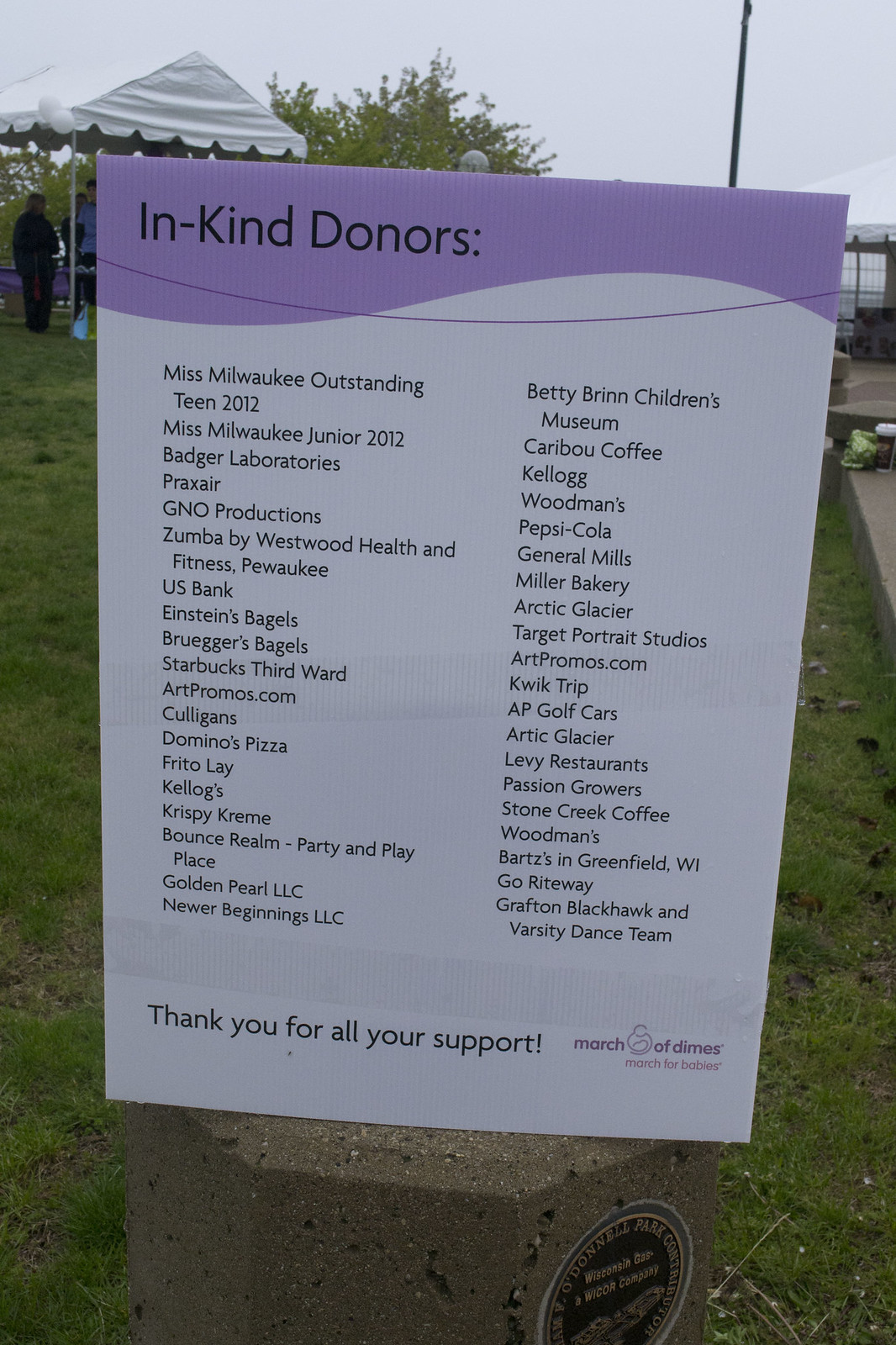The image depicts an outdoor scene featuring a large informational sign set on a rock pedestal or metal stand, situated in a grassy area. The sign has a purple background and prominently displays the words "In Kind Donors" at the top. Below this heading, there is an extensive list of donors, arranged in two columns. The left column includes names such as Miss Milwaukee Outstanding Teen 2012, Miss Milwaukee Junior 2012, Badger Laboratories, Praxair, GNO Productions, Zumba by Westwood Health and Fitness, U.S. Bank, Einstein's Bagels, Bruegger's Bagels, Starbucks Third Ward, ArtPromos.com, Culligan's, Domino's Pizza, Frito-Lay, Kellogg's, Krispy Kreme, Bounce Realm, Party and Play Place, Golden Pearl LLC, Newer Beginnings LLC. The right column contains additional supporters including ArtPromotions.com, Quick Trip, AP Golf Cars, Arctic Glacier, Levee Restaurants, Passion Growers, Stone Creek Coffee, Woodman's, Bart's in Greenfield, Wisconsin, Go Right, Grafton Blackhawk, and the Varsity Dance Team. At the very bottom of the sign, it says "Thank you for all your support," with a mention of "March of Dimes, March for Babies" in the right-hand corner. The background of the image shows a gray overcast sky, a part of a tree, some distant people, and possibly the top of a tent or awning.